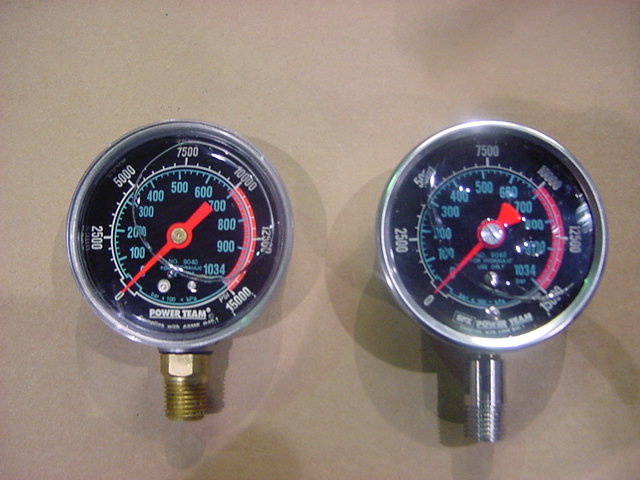In the image, there are two power tram gauges positioned side by side, each characterized by circular faces featuring distinct demarcations. Both gauges have a red needle at their center. The inner circle of each gauge, marked in light blue, displays numbers ranging from 100 to 1034 in a clockwise direction. Surrounding this inner circle, white numbers are visibly marked at intervals from 0 to 15,000. 

Each gauge has an extension protruding from its bottom. The extension of the left gauge is brass-colored and threaded, suggesting it can be screwed onto another component. The right gauge, although slightly out of focus compared to the left, has a nearly identical design except for its silver-colored base. The left gauge is sharply detailed, allowing easy readability, while the right gauge's slight blur and silver base differentiate it.